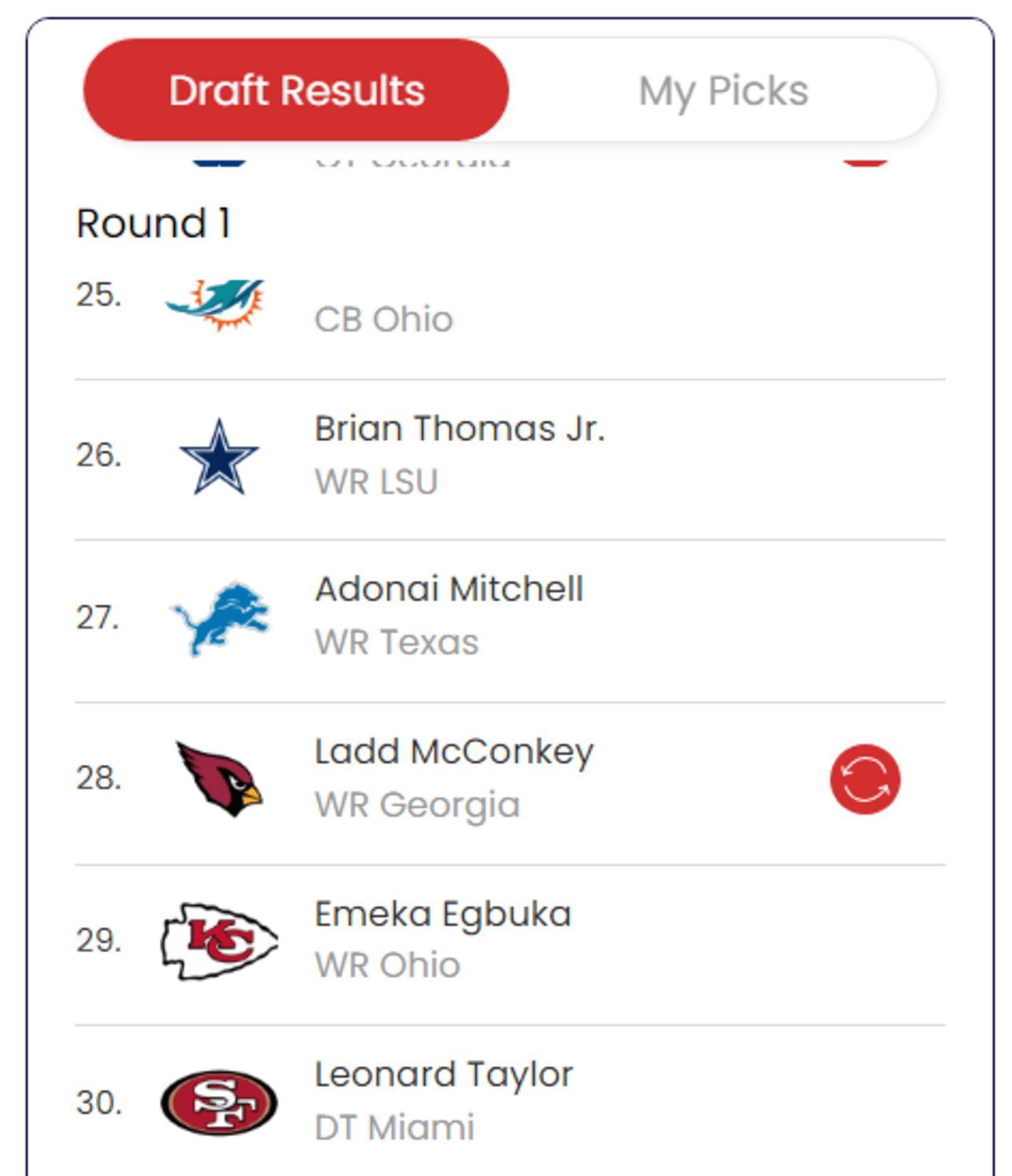Detailed Caption:

In this image, we see a digital draft results page for the NFL, designed for avid fans who keep a keen eye on the rankings of NFL draft results. The draft results are prominently displayed in red. The page is titled "Draft Results" under which it indicates "Round One" with a list of teams and their corresponding picks.

At the 25th position, the Miami Dolphins have picked a player from Ohio State. The Dolphins' logo features a blue dolphin within an orange circle. 

The 26th pick is Brian Thompson Jr., a wide receiver from LSU. 

Following him, at the 27th position, the Detroit Lions selected Adonai Mitchell, another wide receiver, this time from the University of Texas.

In the 28th position, it lists Ladd McConkey, a wide receiver from Georgia, next to an icon with two circular arrows indicating a potential repeat or exchange.

At position 29, the Kansas City Chiefs have picked Emeka Egbuka, a wide receiver from Ohio State.

Lastly, at position 30, Leonard Taylor, an interior defensive tackle (IDT) from Miami, rounds out the visible draft selections.

The background of the page is white, and above the "Round One" title, a portion of the header appears cut off, possibly indicating another section or team information that is not legible in this image. This captures a snapshot of the frenetic but highly organized NFL draft process, highlighting the excitement and anticipation of adding fresh talent from college teams to professional rosters.